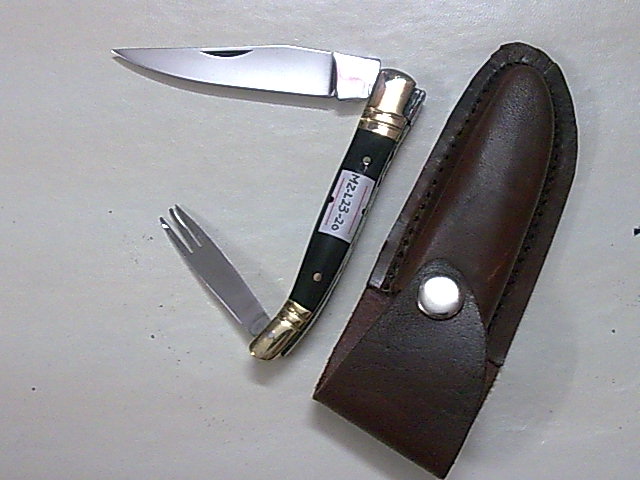The image depicts a meticulously well-maintained pocket knife and its corresponding sheath. The knife, predominantly black with silver ends, is partially opened, revealing a dual-purpose design. One end features a sharp, silver blade, approximately 2.5 inches long, while the opposite end intriguingly displays a three-pronged fork, hinting at a versatile utility. The handle sports a white square label marked with the serial number "MZL23-20," suggestive of an identification tag or price marker. This pocket knife rests on a neutral background—appearing either gray or white—providing a clear, unobstructed view of the items. Beside the knife lies its meticulously crafted dark brown leather sheath, secured with a silver snap button. The sheath remains closed, displaying an elegance that complements the knife's pristine condition, reminiscent of either a collector's display piece or a finely preserved item in a specialty store.